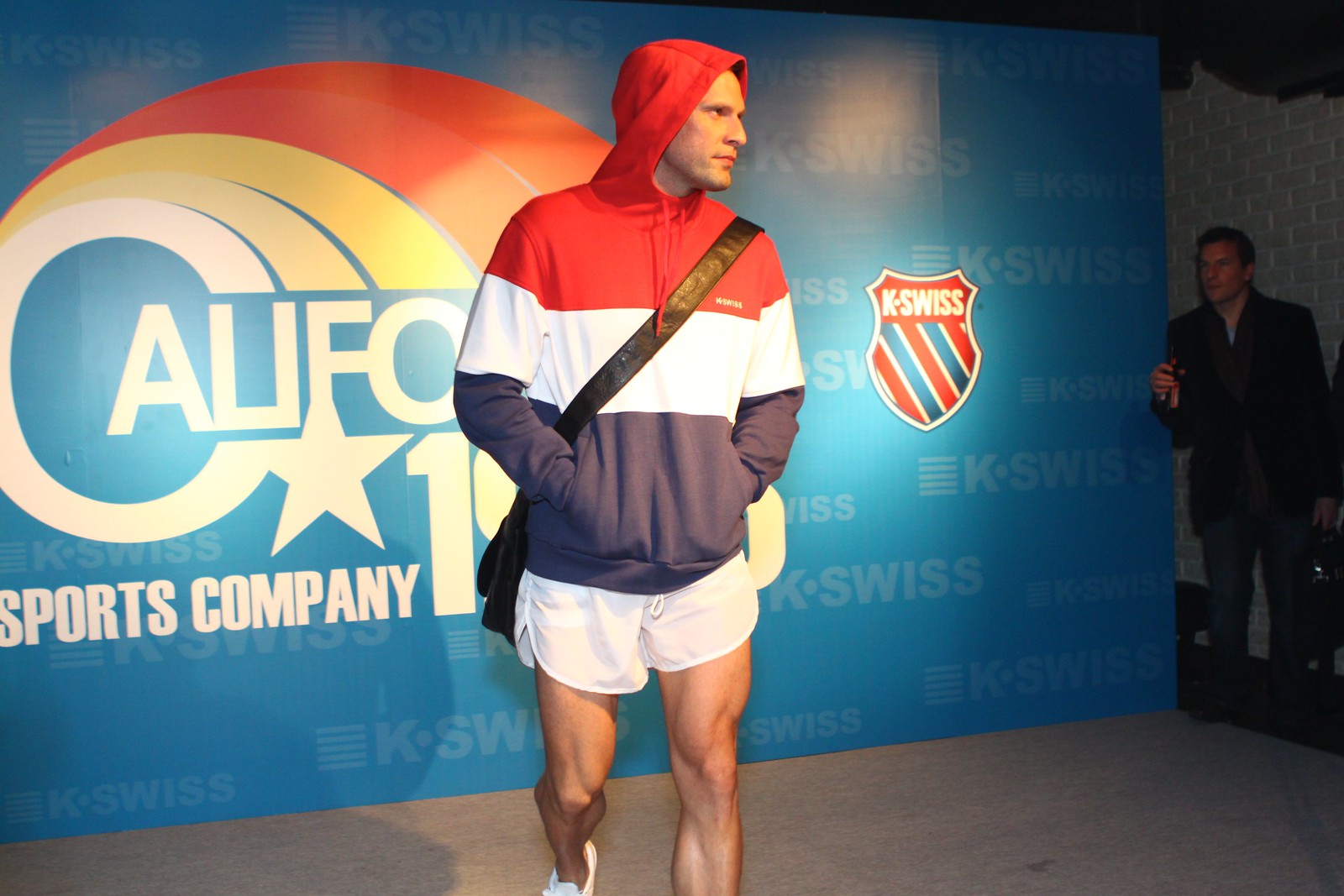In this image, there is a sports player prominently positioned in front of a large blue sign that is covered with the K-Swiss logo, featuring a red and blue shield design with blue stripes. The sign behind him also includes the word "California" and a star, followed by the phrase "sports company." The athlete is dressed in white shorts, displaying muscular legs, and white tennis shoes. He also wears a long-sleeved hoodie with red, white, and blue stripes, with the hood up. Over his shoulder, a black bag hangs down toward his hip, and he has his hands in his pockets while looking to the left. On the far right of the image, a man in a black jacket holds a microphone and looks on. This scene appears to be a promotional or modeling event for K-Swiss sports apparel.